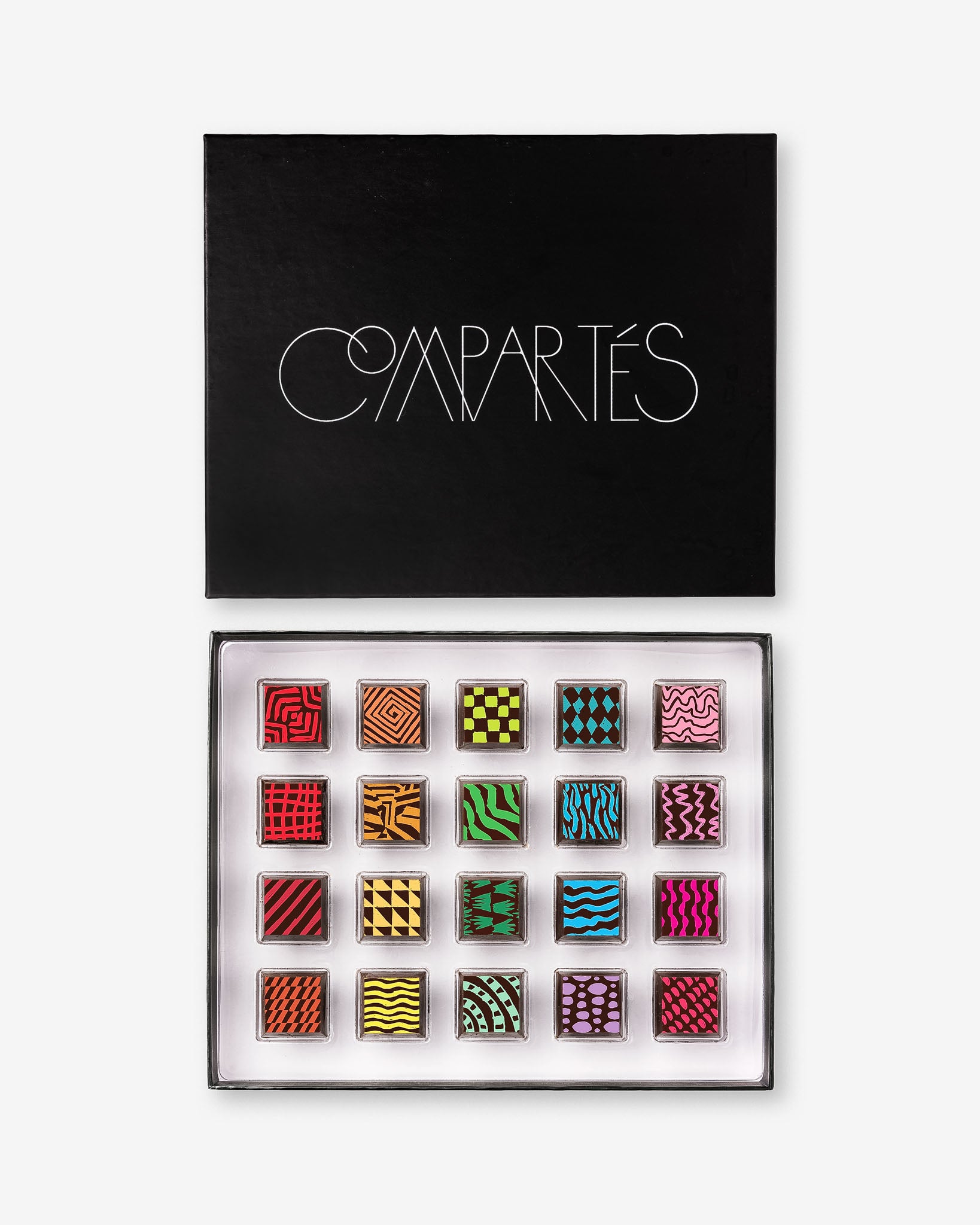In front of me is a color photograph of an open display case set against a pale gray background. The display case features a black lid laying flat, printed with the word "Compartés" in capital letters—the 'E' adorned with an accent mark. Below the lid, the inside of the display case is arranged neatly with four rows of five colorful squares, each nestled in a white tray, framed by a black backdrop. These squares come in an array of striking neon colors including red, black, green, orange, blue, and pink. Each square is uniquely adorned with different patterns such as checkered designs, waves, squiggles, check marks, diamond shapes, tigers, dashes, and triangles. The vivid, diverse designs and vibrant hues create a visually captivating and colorful display.